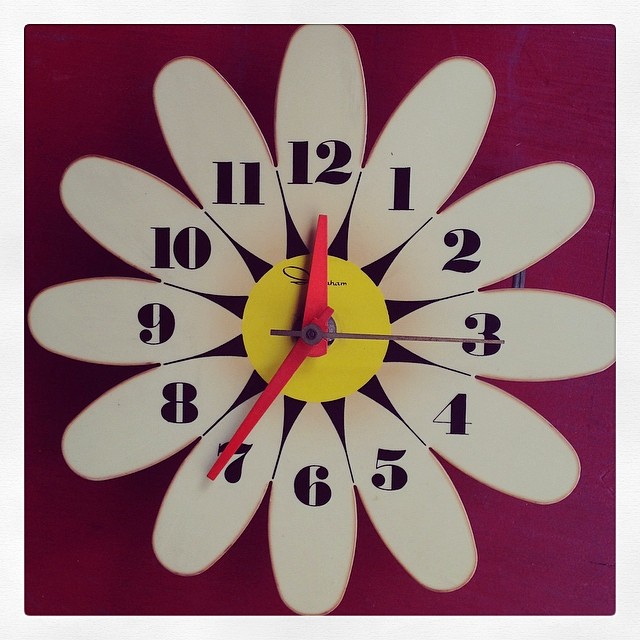This image features a striking square clock set against a vibrant red background. Notably, the clock itself is also square-shaped, creating a harmonious visual symmetry. The clock face is adorned with black numbers that uniquely run counterclockwise, beginning with one at the top. These numbers are thoughtfully arranged in a floral pattern, with each number positioned on a white petal-like shape. At the center of this floral design is a sunny yellow circle, adding an eye-catching focal point. The clock's hands are vivid red, with an additional brown hand for further detail. There is also visible writing on the clock, though the specific text is not clearly readable in the image.